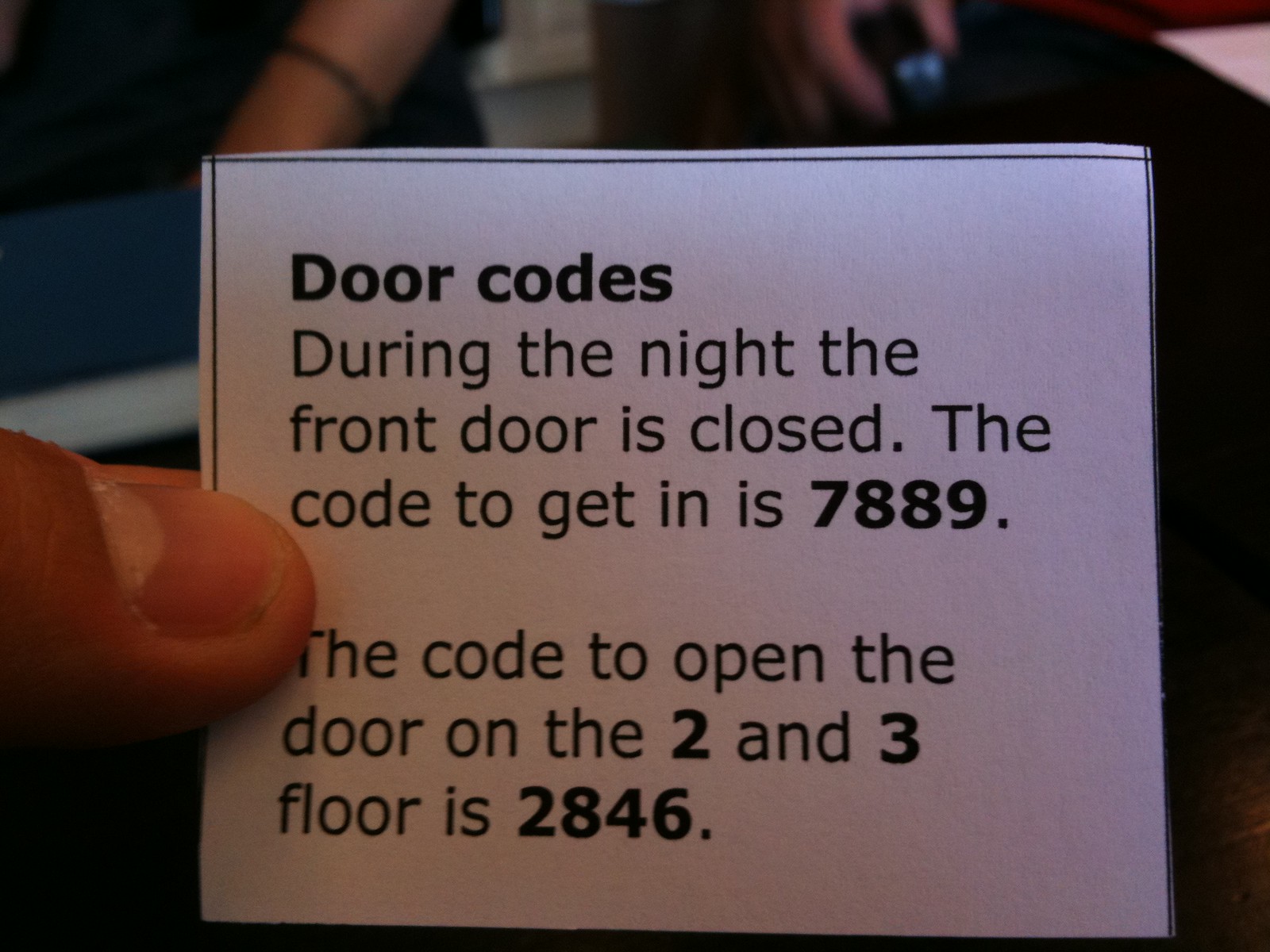The image displays a close-up of a small white card with black text held between a person's fingers. The card's text, titled "Door Codes" in bold, details entry codes for a building. Specifically, the night code for the front door is "7889," and the codes for the second and third floors are "2846," with all numbers also in bold. The hand holding the card emerges from the left side, positioning the card prominently in the center of the image. The scene's background, though blurred, reveals faint shapes of individuals seated around a table, contributing to a setting that suggests an indoor environment with these door access instructions. The overall color palette includes white, black, beige, blues, reds, grays, and tan.